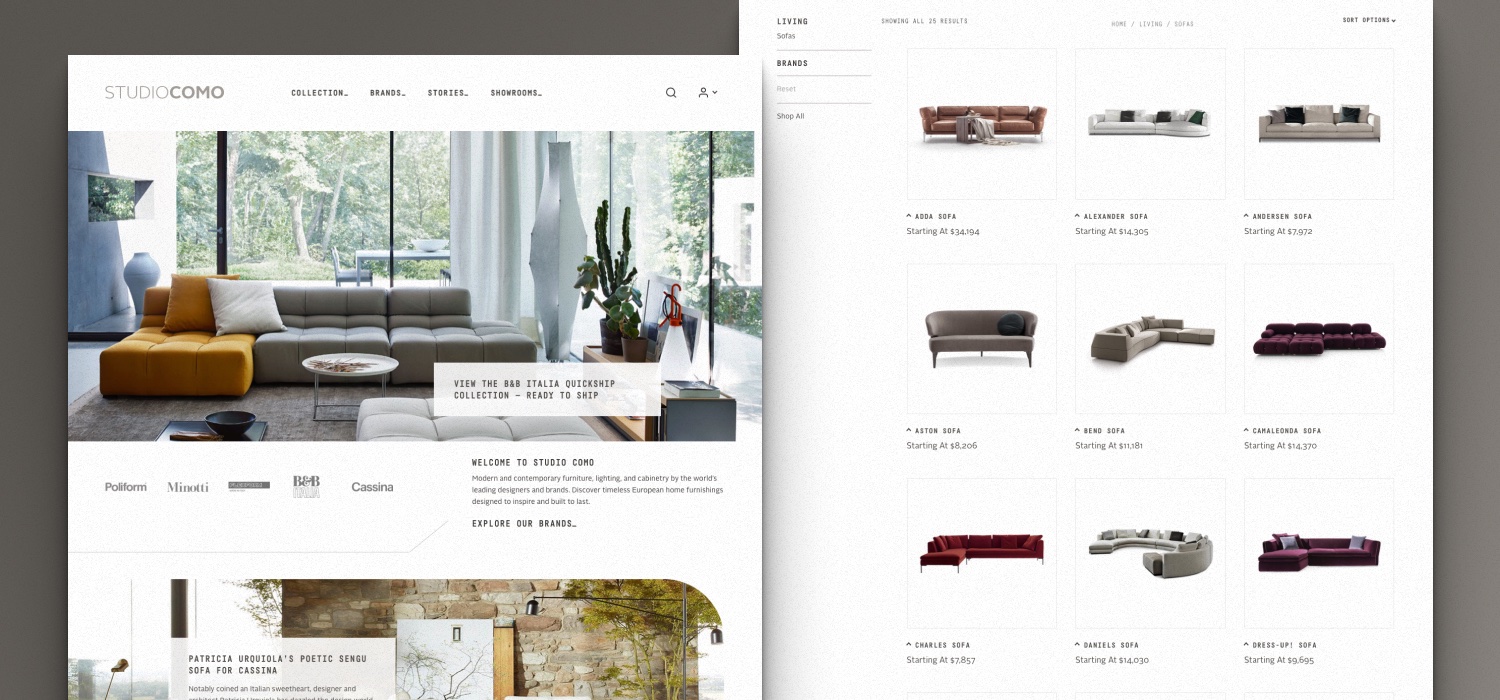The website features an innovative, book-like design that showcases furniture collections. On its left side, a dark gray band adorns the border, running vertically along the edge and horizontally across the top, with the name "Studio Como" prominently displayed. The primary section on this page includes a photograph depicting an elegantly arranged furniture setting, followed by descriptive text offering insights and details. Adjacent to this, another photograph occupies the lower section but is partially cut off, seamlessly flowing to the adjacent page.

On the right, a complementary dark gray border mirrors the left, framing a series of sofa images. Each sofa is set against a crisp white background, highlighting different styles, colors, fabrics, and pillow arrangements. Accompanying each sofa image is its title and starting price, providing clear and organized information for potential buyers. The overall page layout is minimalist yet informative, emphasizing the beauty and variety of the showcased furniture.